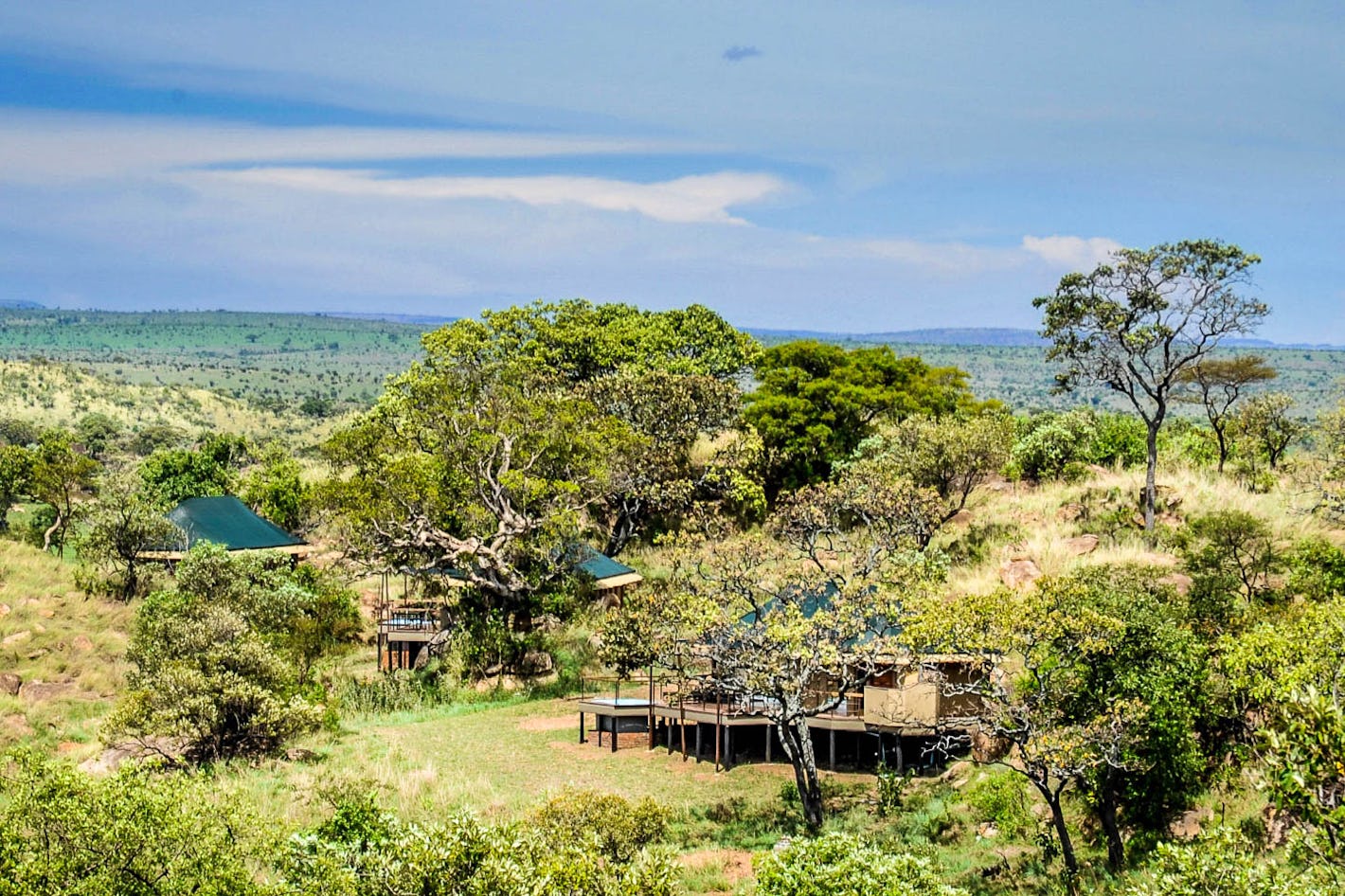The photograph captures a mid-day scene of a small, secluded encampment nestled among the hills, likely in the Serengeti. The area is heavily frosted with lush, green foliage interspersed with a variety of trees spreading out to the horizon, accompanied by sagebrush. Three distinct houses on stilts are built into the side of the hill, each featuring slanted green roofs, which might house solar panels, and large, metal-railed decks. The structures appear modern and newly built to withstand marshy conditions. One of the houses closest to the foreground even has a visible pool. The ground below the houses is lush and green, creating an illusion as though the buildings are floating in the air. In the background, beyond the basin of the hill, the landscape opens up to a large valley covered with dark green grass, leading up to a bright blue sky streaked with elongated white clouds. The entire setting exudes the feel of a serene, isolated resort area amidst a vibrant natural landscape.